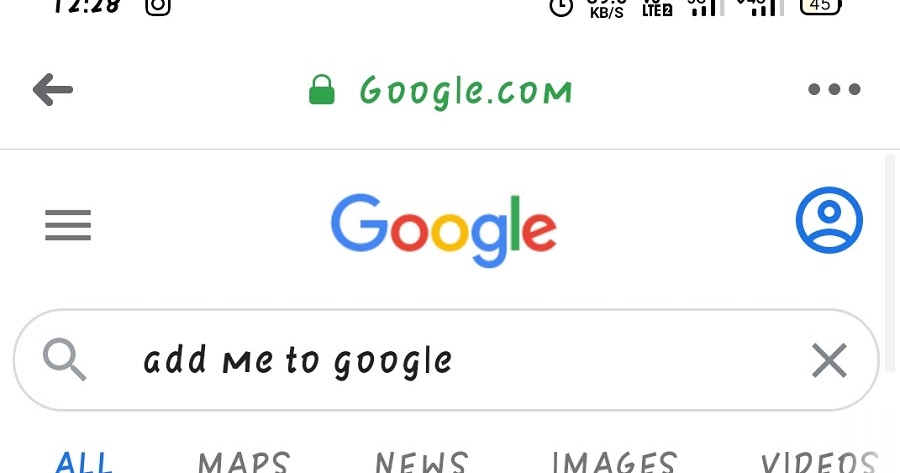This screenshot captures a web page referencing Google.com. Centered at the top is the URL, "Google.com," elegantly displayed in a green typewriter-style font, accompanied by a green padlock icon, indicating a secure connection. The current time is shown as 12:28, and the Wi-Fi signal icon suggests an active internet connection. The battery level is visible at 45%. Beneath the URL are navigation options: a left arrow button, three gray dots, and three stacked gray lines, possibly for additional settings or menus.

Prominently featured is the colorful Google logo with the letters "G" in blue, "O" in red, the second "O" in yellow, "G" in blue, "L" in green, and "E" in red. Below the logo, there's a prominent search bar with the text, "Add me to Google," and a small "X" button within the search field. Further navigation links are provided for "All," "Maps," "News," "Images," and "Videos," offering a comprehensive guide to different types of search content available.